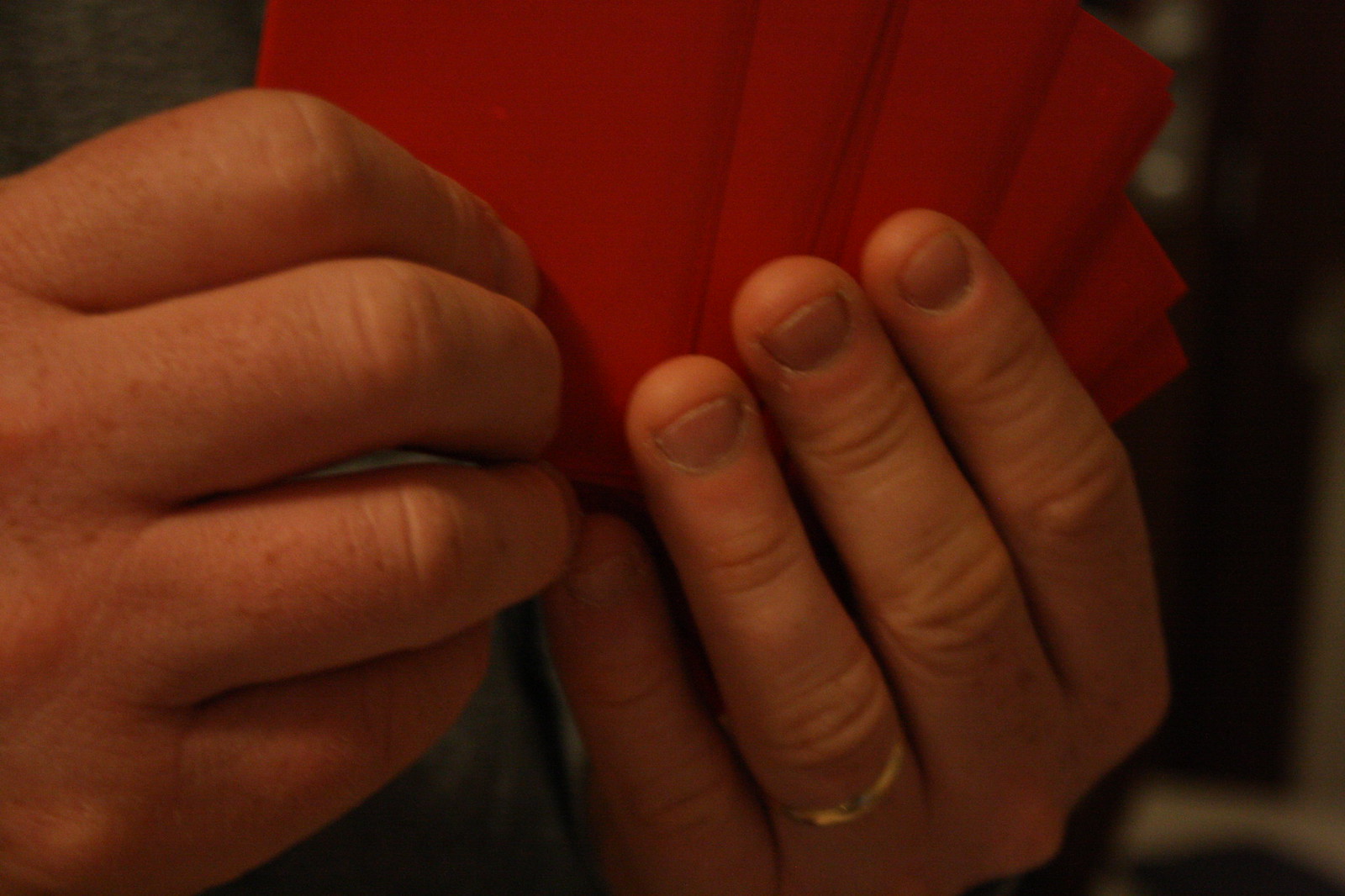In this close-up image, we see a person's large hands, likely a man's, prominently holding a fan of red cards. The individual's hands, characterized by thick, short fingers and a gold wedding ring on the left hand, are positioned center-frame, facing forward towards the viewer. The background is predominantly dark and out of focus, though there are a few light sources creating a soft glow, particularly visible through white circles in the upper right corner. The surrounding border of the image transitions from black to a beige-tan hue as it moves towards the bottom. In the upper left and bottom left corners, there are glimpses of a gray fabric, likely the shirt of the person holding the cards. The overall composition directs the viewer's attention to the vividly displayed cards, which, unlike traditional playing cards, feature a plain red design.